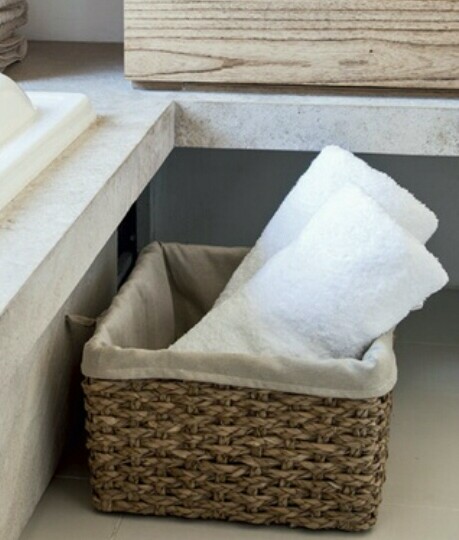The image captures a partial view of an elegant bathroom corner, featuring a countertop that appears to be made from white faux marble. Atop the counter rests a piece of polished wood, possibly serving as a cabinet or storage unit, though its full design is not visible. To the left, there is a neatly stacked set of gray towels, emphasizing the tidy and organized ambiance. Further left, the image reveals the beginning of a pristine white bathtub with a step-down feature, though details like the shower head or faucet fixtures remain obscured. Centered in the image is a stylish brown wicker basket, accented with a pale brown lining that protects its contents. Inside the basket are two immaculately rolled, large white towels, likely intended for bathing rather than hand use. The overall appearance and amenities suggest that this bathroom could belong to a high-end spa or a hotel, designed for guest comfort and luxurious relaxation.